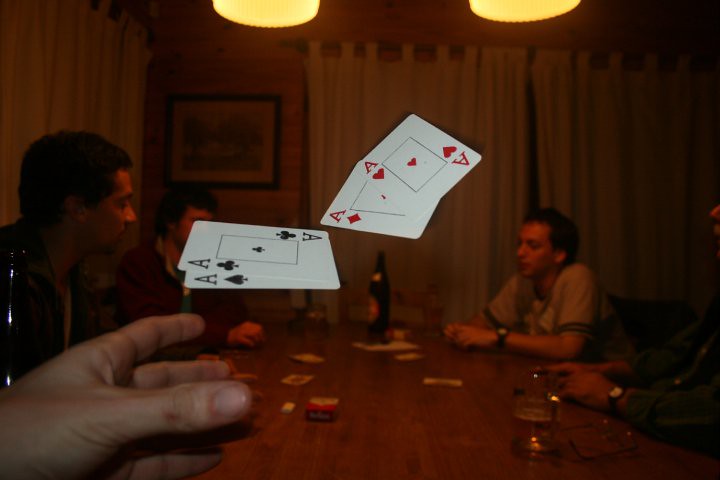In this image, a card game unfolds around a sizable, brown wooden table. At the forefront, from the bottom left corner, a hand is dramatically captured mid-air, having just flung four aces – clubs and spades on the left, diamonds and hearts on the right. The hand's thumb, underside of the index finger, and middle finger are clearly visible. 

On the left side of the table, a person with short black hair is observed from the side. Behind them, another individual, partially obscured by the airborne cards, wears a red jacket and rests one hand on the table. Centrally placed on the table is a dark brown bottle of beer, serving as the room's focal point.

To the right side, a person wearing a gray t-shirt with black rings on the sleeves is seen from a side angle. Nearby, another individual, whose face is not visible, dons a green jacket and places both hands on the table. The foremost hand also sports a watch. Adjacent to this individual, a half-filled glass is noticeable.

Scattered on the table are a red, black, and white pack of Marlboro cigarettes and several miscellaneous playing cards. The setting appears to be a dimly lit living room, evidenced by white window curtains in the background. The room is illuminated by two overhead lights, while a square black picture frame with a white image inside hangs on the back wall.